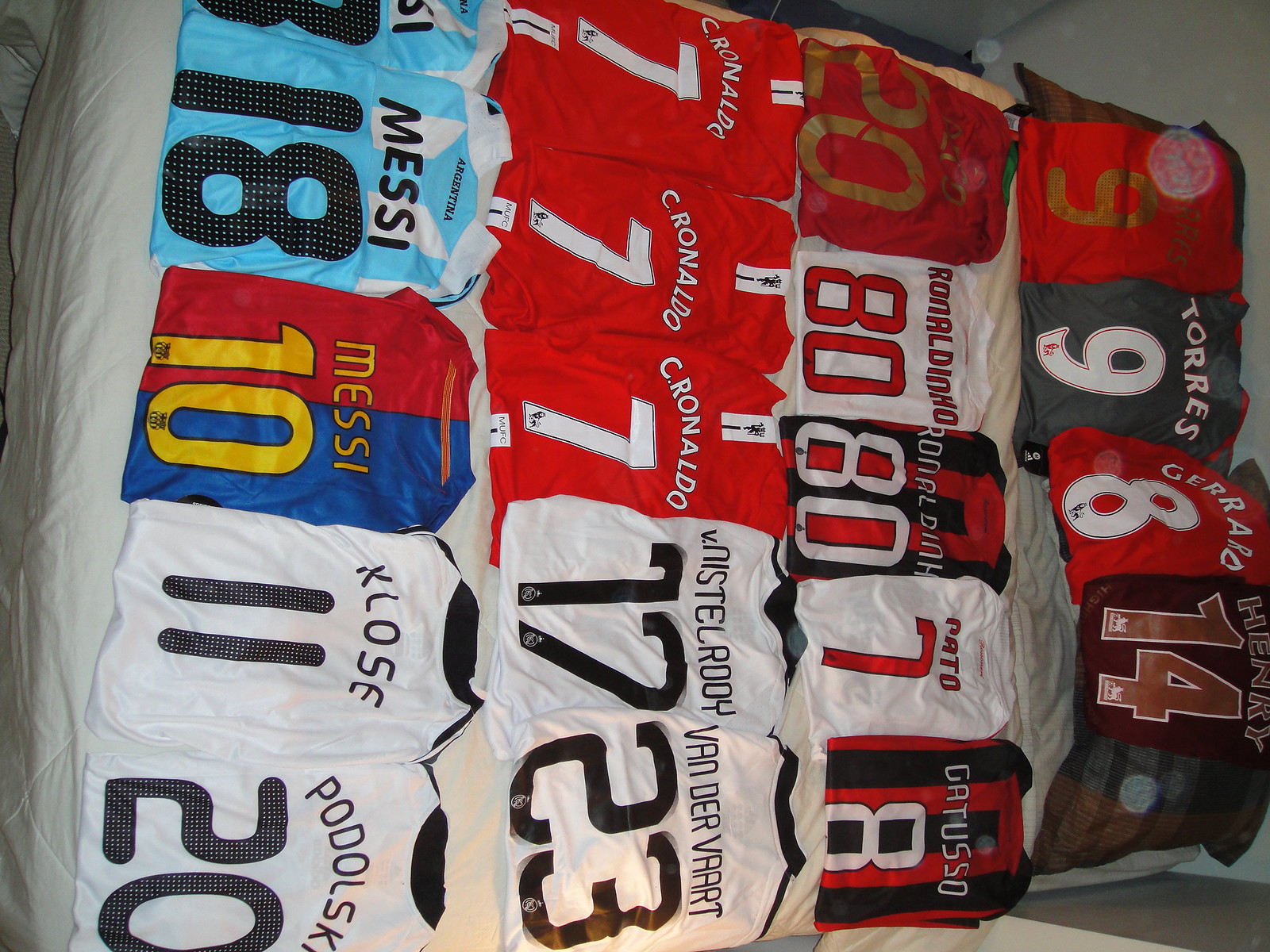This is a detailed, overhead photograph of a bed completely covered in neatly folded sports jerseys, specifically soccer uniforms. The jerseys are organized in four rows, each facing left in the image, and showcase an array of vibrant colors including red, black, gray, blue, and yellow. The jerseys prominently display various player names and numbers: multiple "Torres" jerseys with the number 9, "Ronaldo" with number 80 in different colors, "Gerard" with number 8, "Henry" with number 14, "Gattuso" with number 8 in black and red, "Messi" appearing several times with numbers 10 and 18, "Klos" with number 11 in white and black, and "Van der Vart" with number 23. The uniforms come in a variety of color schemes, including light blue, red and blue, and white with red letters, adding to the visual appeal of the collection.